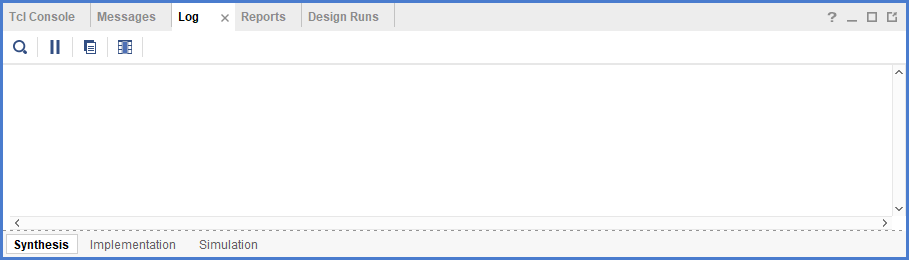The image depicts a computer screen displaying a software interface in landscape orientation. The interface is divided into various sections, each containing specific functions and options. 

At the top of the screen, there is a narrow toolbar with quick access options such as "TCI Console," "Messages," "Log," "Reports," and "Design Runs." On the right side of this toolbar, there are several icons, including a question mark for help, a minimize button, an open file icon, and an additional, unidentified icon.

Below the top toolbar, on the left side, there is a vertical strip of icons including a search icon, a stop icon, and two other unidentified icons. 

The main area of the screen is currently displaying the "Log" page, which is completely empty, indicated by the lack of any visible data or entries on the page. The screen also features scroll left and right arrows, as well as scroll up and down arrows, which suggest that the page could be navigated if there were any content to display.

At the bottom of the screen, there are three tabs labeled "Synthesis," "Implementation," and "Simulation." The "Synthesis" tab is currently selected, as indicated by its bold and white appearance, while the other two tabs are grayed out.

Overall, the visual elements and interface suggest that the user has navigated to the "Log" page within the "Synthesis" section and found no entries or data to display.